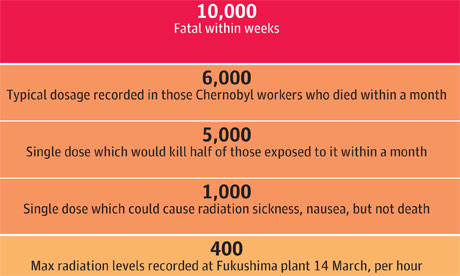The image features a detailed chart composed of five horizontal bars, each varying in color intensity from a deep red at the top to a pale yellow at the bottom, illustrating the lethal effects of radiation dosages. The topmost bar, colored in deep red, is marked with "10,000" in white text, indicating a fatal dose within weeks. Below it, three consecutive orange bars are displayed. The first orange bar reads "6,000" in black, denoting the typical dosage recorded in Chernobyl workers who died within months. The second orange bar is labeled "5,000," representing a single dose that would kill half of those exposed within a month. The third orange bar shows "1,000," indicating a single dose that could cause radiation sickness and nausea but not death. The final bar, colored in mango yellow, is labeled "400," describing the maximum radiation levels recorded at the Fukushima plant on 14 March, per hour.